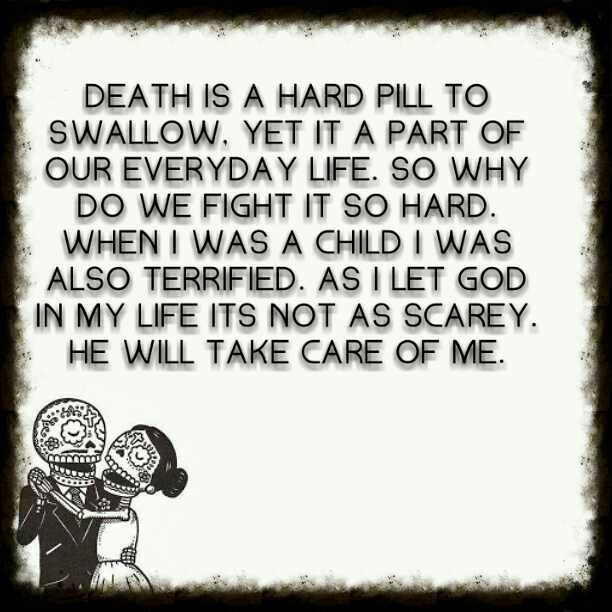The image is a black-and-white illustration with a distinctive black border that fades into a fuzzy, irregular edge. In the bottom left corner, there are two animated skeleton figures dancing together. The skeleton on the left appears to be male, adorned in a tuxedo, while the one on the right is female, dressed elegantly with hair styled in a bun. Both skeletons feature intricate designs on their skulls, including flowers and crosses, and they are depicted smiling and holding each other as they dance. The upper portion of the image contains a centered, bold text in all caps that reads, "Death is a hard pill to swallow, yet it is a part of our everyday life, so why do we fight it so hard? When I was a child, I was also terrified. As I let God into my life, it is not as scary. He will take care of me."